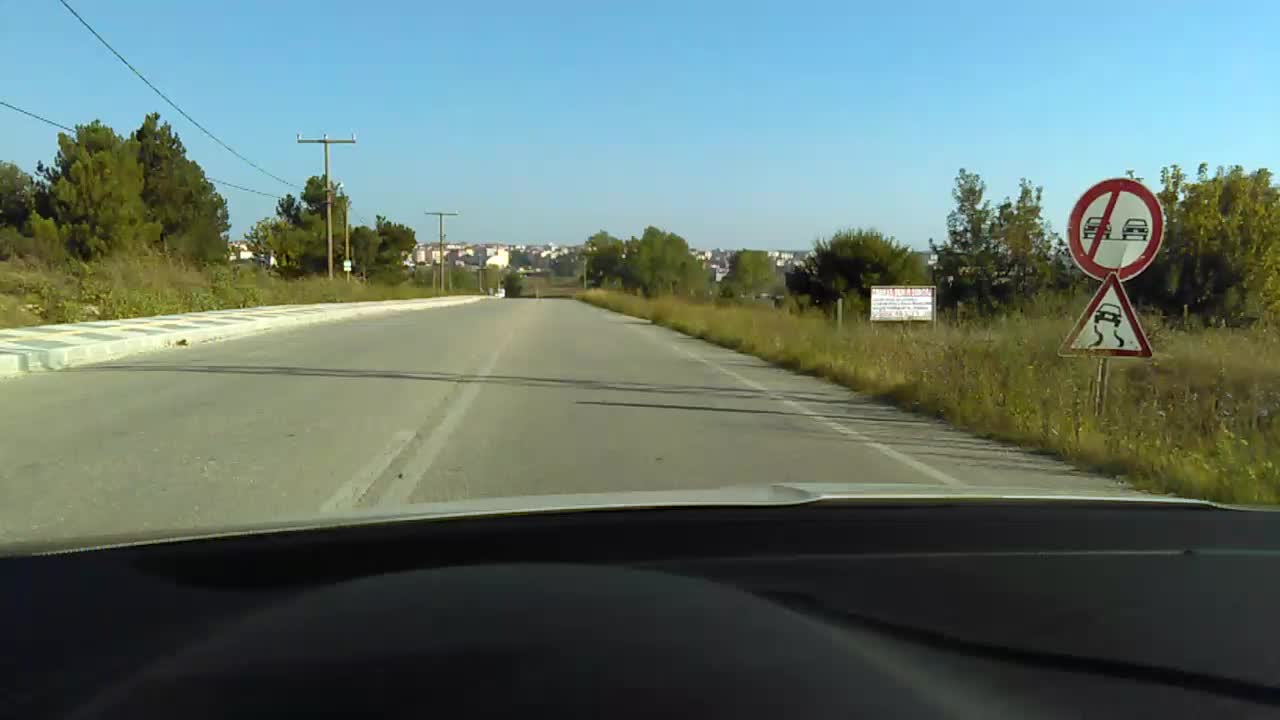This image provides a view from inside a car, possibly taken by a dash cam, looking out onto a calm, empty road during the daytime. The scene is set on a country or suburban road with a clear blue sky and no visible traffic or pedestrians. On the right-hand side of the road, there are two prominent traffic signs. The first sign, a circular one with a line through two cars, indicates a no-passing zone. The second sign is a triangular warning sign with a depiction of a car and skid marks, suggesting caution for an uneven or possibly slippery road ahead. On the left side of the road, there is vegetation including shrubs and trees, and telephone poles lining the route, adding to the landscape's suburban feel. The road itself has faded white painted lines, hinting at wear. In the background, buildings suggest a small town or residential area, and the dry landscape hints at a warm climate. The calmness of the scene, with no vehicles or people in sight, emphasizes the tranquility of this journey.